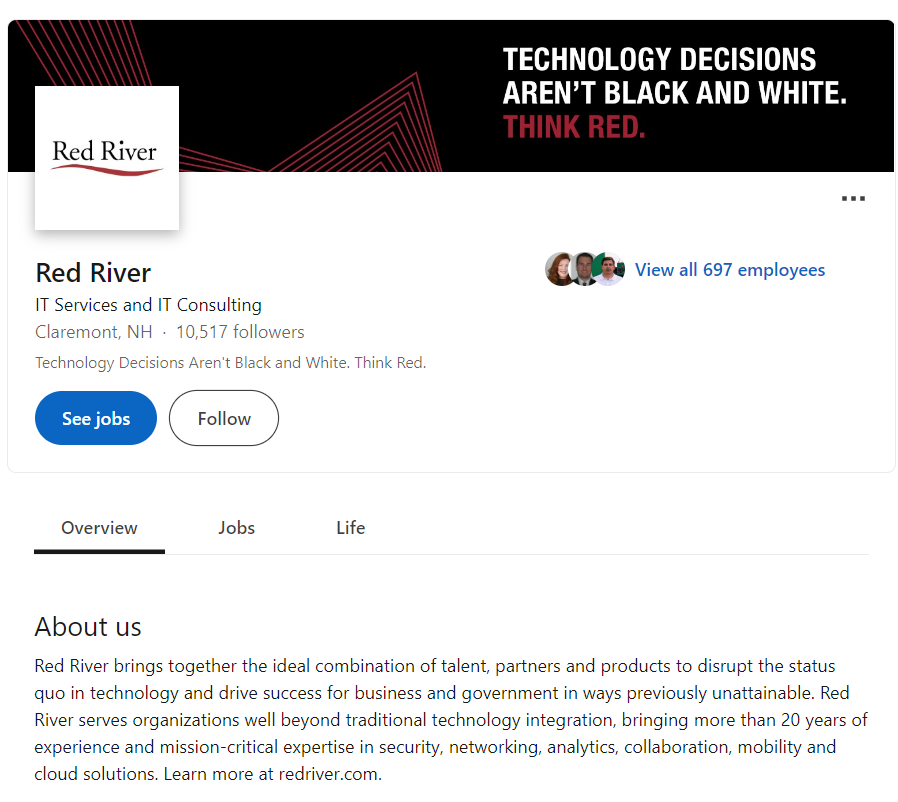The image appears to be a webpage from a job search website, likely similar to platforms such as Indeed, Glassdoor, or LinkedIn. The page displayed is dedicated to a company named Red River. At the top, there is a small banner featuring the company's slogan: "Technology decisions aren't black and white, think red." The phrase "think red" stands out in red text, while the rest is in white, set against a black background with red geometric lines for decorative effect.

Beneath the banner, the company's logo is prominently featured. The logo consists of the text "Red River" in bold, black letters with a red underline resembling a ribbon. A brief profile of the company follows, describing Red River's services as specializing in IT Services and IT Counseling, and indicating that the company is based in Claremont, with 10,517 followers.

The slogan "Technology decisions aren't black and white, think red," is reiterated below this information. To the right, there are three small photos of employees with an adjacent link in blue text that says "View all 697 employees." In the same section, there are also two buttons: a blue "See Jobs" button and a white "Follow" button.

Further down the page, the layout shifts to tabs labeled "Overview," "Jobs," and "Life," with the "Overview" tab currently selected. This section offers a brief description about the company under an "About Us" heading, providing potential job seekers with more information about Red River's mission and values.